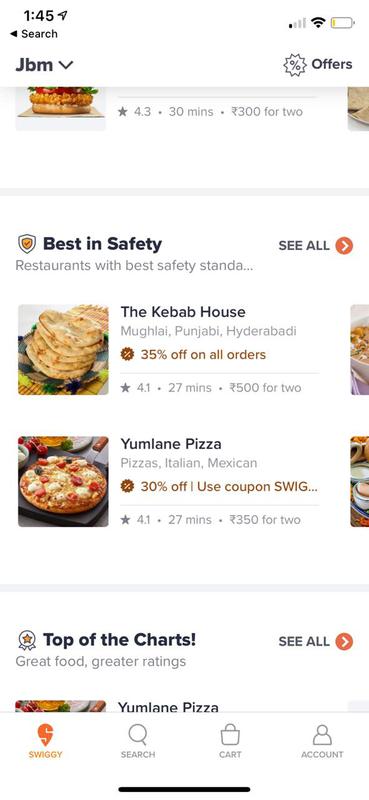The image is a mobile interface, possibly from a food delivery app, loaded with various icons, symbols, and text details. Here is a cleaned-up and detailed caption:

---

At the top of the screen, the status bar reads "145" next to an icon resembling a paper airplane. Following that, there are four lines of varying lengths with the first one in black and the remaining three in gray, likely representing signal strength. The Wi-Fi symbol and a battery indicator with a small yellow segment are also present. Below, the text reads "JMB" with an arrow pointing downward.

A starburst icon labeled "Offers" is displayed, followed by a partial image of some food item. Adjacent to this is a star icon in gray labeled "4.3," followed by a dot, and the text "30 minutes." The text “$2300 for 2” or "$3 for 2" is unclear. The phrase "Best in Safety" is accompanied by a shield-like symbol containing a yellow area with an orange checkmark. 

The text “See All” appears next to an orange circle with a right-facing arrow. Underneath, the phrase "Restaurants with the Best Safety Standa…" is partially cut off. "The Kebab House" is listed, accompanied by an image that appears to be pita bread with some unclear text below it. Another starburst icon indicates "35% off on all orders" with a rating of "4.1," "27 minutes," and the text "$5 for 2."

An image of a pizza is captioned "Yumling Pizza, Pizza Italian Mexican," accompanied by a starburst indicating "30% off" with the coupon code "SWIG…" visible. Ratings show "4.1," "27 minutes," and "$3.50 for 2." Below is a gray bar with the text "Top of the Charts." To its left is an award-like symbol, and to the right, "See All" is written with an orange circle and a right-facing arrow. 

Just visible is the top of "Yumling Pizza" branding, stylized as an orange "S" with yellow writing. At the bottom, icons for "Search" (magnifying glass), "Cart" (bag), and "Account" (head and shoulders outline) are present, with a black line underneath them.

---

This caption clearly describes every element of the interface, making it easy to visualize the layout and contents.